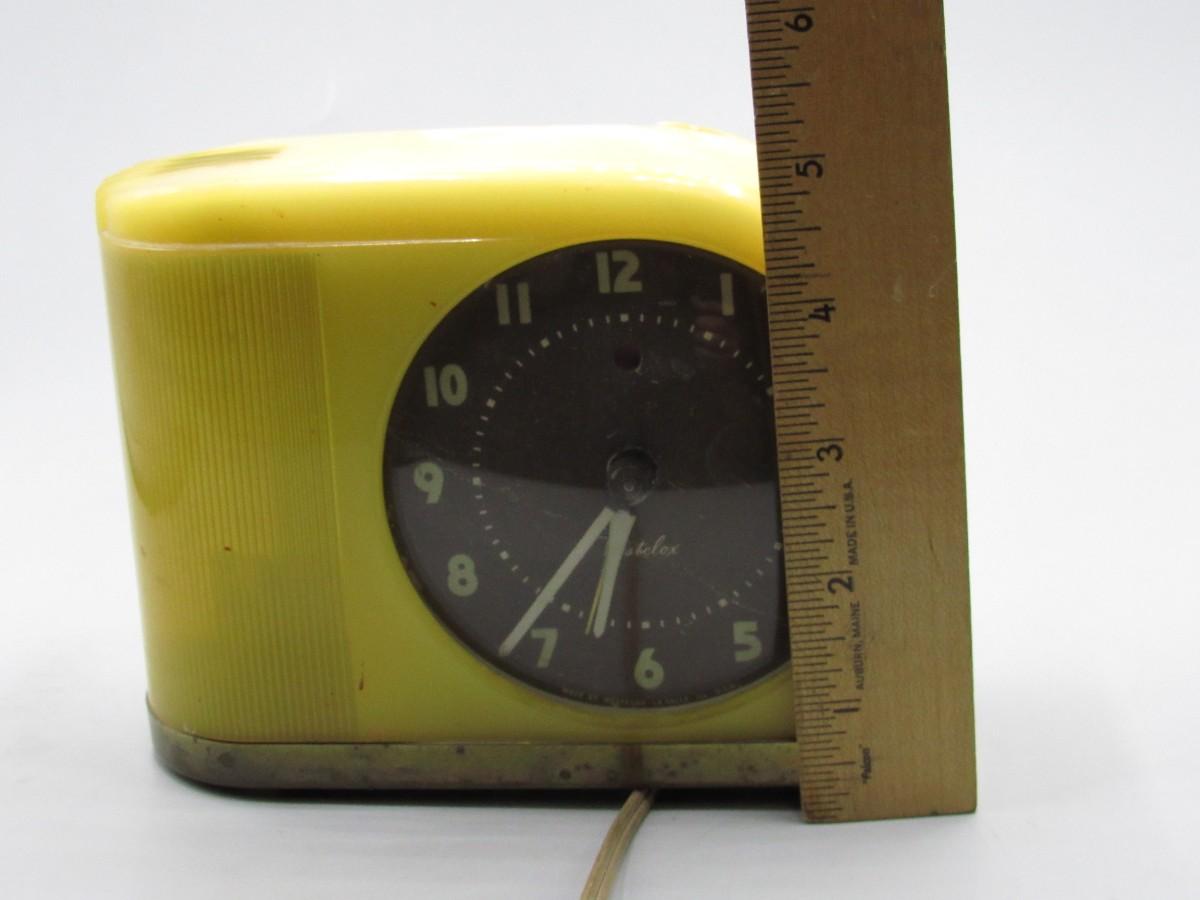This photograph features a vintage-style, yellow plastic desk clock with a black analog face showcasing white numbers (1 through 12) and hands indicating the time at approximately 6:41. The clock measures about five inches in height, as indicated by a wooden ruler standing vertically next to it. An off-white power cord emerges from beneath the clock, which rests on this cord. The background of the image is an off-white color, providing a neutral contrast to the clock’s vivid yellow casing and its black face.